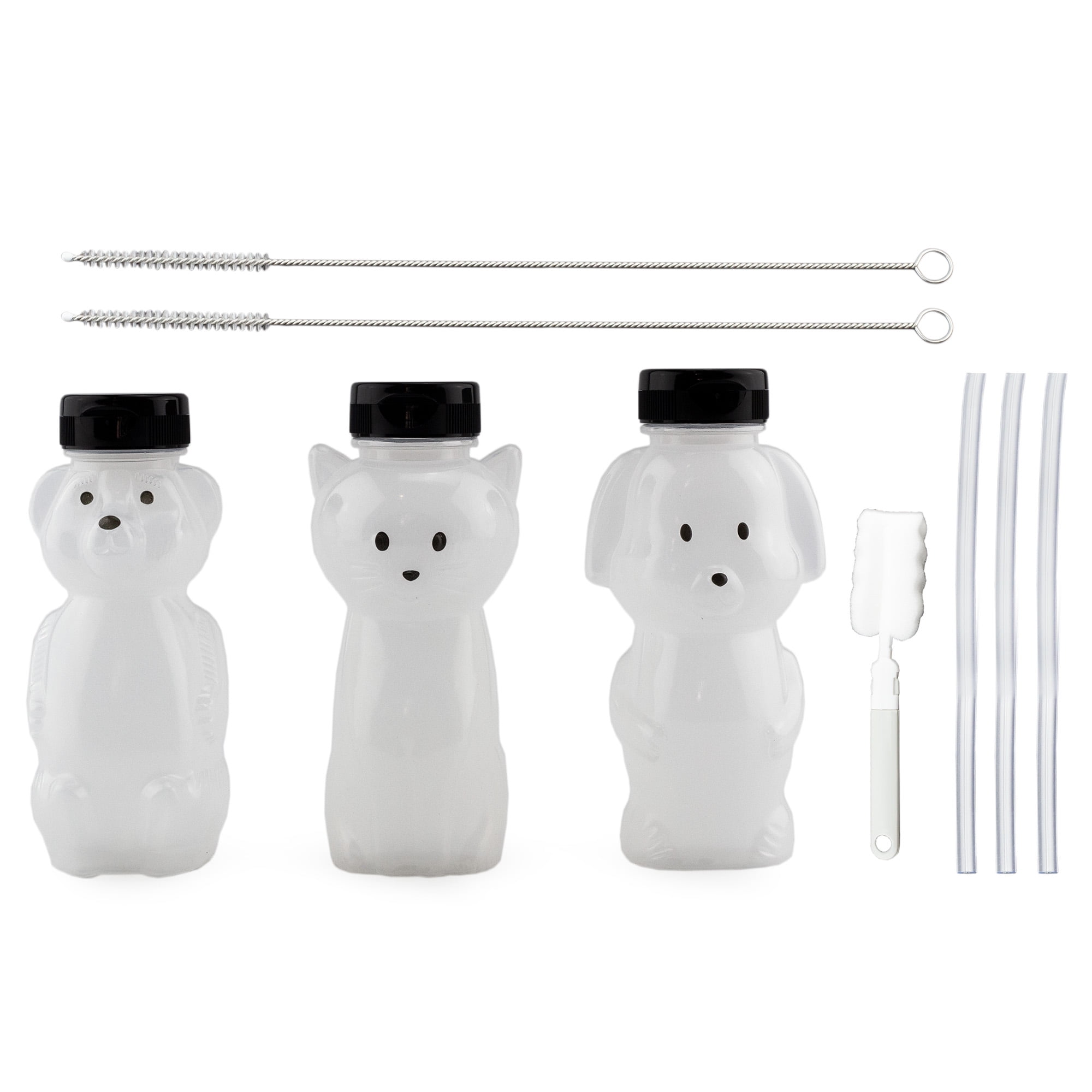The photograph on a white background features three plastic bottles shaped like animals: a bear on the left, a cat in the center, and a dog on the right. Each bottle is white with black dotted eyes and noses, and they are capped with black lids. Above them are two identical cleaning brushes with wire handles forming a circular loop at the ends. To the right of the dog bottle, there is another plastic brush with a white head and handle, positioned vertically. Further to the right, there are three white straws. The image appears to showcase these items, likely intended for purchase, arranged neatly against a stark white setting, with no date or text included.